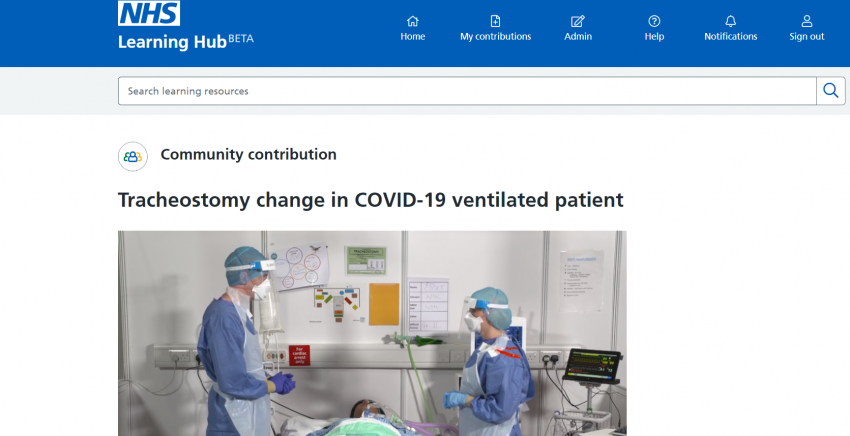The website features a header in a rich royal blue color. On the left side of the header, there is a logo consisting of the white letters "NHS" set against a blue rectangular background. Below the logo, the text "Learning Hub" is displayed in white font. In the upper right corner of the logo, the word "Beta" is presented in a light blue font. 

To the right of the logo, the standard header navigation items, all in white, are lined up: Home, My Contributions, Admin, Help, Notifications, and Sign Out. Directly below the header is a long search box with a magnifying glass icon on its right side.

The main section of the webpage has a white, or possibly a very light blue, background. Above the main headline, the phrase "Community Contribution" is prominently displayed. The main headline, bolded for emphasis, reads "Tracheostomy Change in COVID-19 Ventilated Patient."

Beneath the headline is a photograph of a hospital room. The image captures a man on the left and a woman on the right, both wearing caps, masks, surgical gowns, blue gloves, and aprons. They are fully equipped in protective medical attire. At the very bottom of the photo, a green blanket is visible, covering the patient, and part of the patient’s head can be seen peeking out slightly.